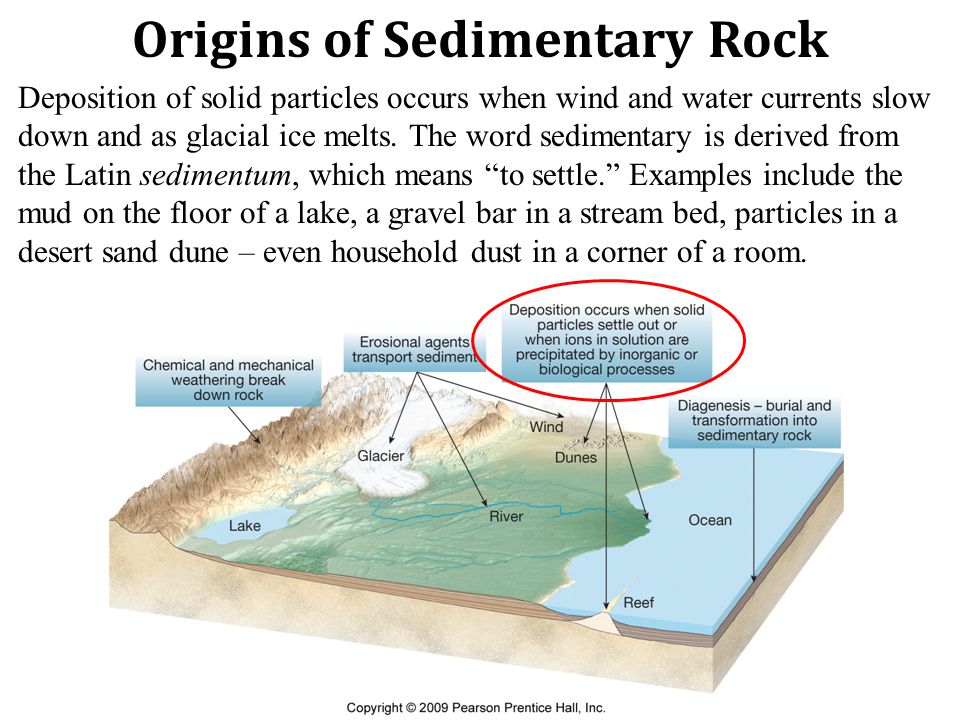The image is a detailed educational PowerPoint slide titled "Origins of Sedimentary Rock" in black text at the top. Below the title, a paragraph explains that the deposition of solid particles occurs when wind and water currents slow down, and as glacial ice melts. It highlights that the word 'sedimentary' is derived from the Latin word 'sedimentum,' meaning 'to settle.' The paragraph also provides examples such as mud on the floor of a lake, a gravel bar on a stream bed, particles on a desert sand dune, and household dust in the corner of a room.

Below this explanatory text, there is a detailed, color-coded topographical 3D map displaying various geological features like mountains, oceans, reefs, rivers, lakes, glaciers, winds, and dunes. Each feature is clearly labeled and corresponds to different sedimentary processes. The colors used in the map include white, black, blue, brown, and green, enhancing the visual distinction between different geographical and sedimentary features. The text is positioned at the top of the slide, while the illustrative map occupies the bottom portion, providing a comprehensive visual aid to the accompanying information.